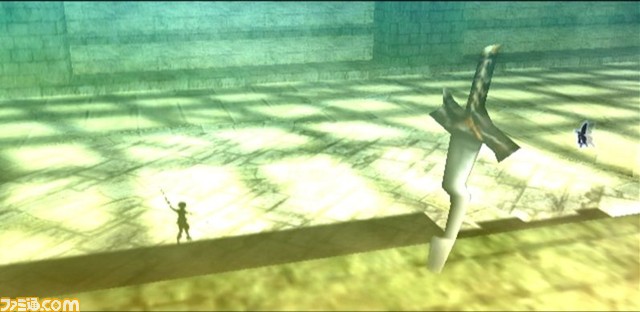The image depicts a fantasy scene from a digital or video game with a cartoon-like aesthetic. In the background, a large cobblestone wall emanates a greenish hue, with an open section of slightly different color suggesting an entrance or archway. The ground comprises intricately patterned large rock tiles, reminiscent of Aztec designs. A lush grassy area occupies the foreground.

Dominating the scene is a gigantic sword embedded in the ground, towering like a skyscraper with a unique design: a square section cut out of the middle of the blade, a dark gray hilt, and handle. To the left stands a small, brown character, silhouetted and holding a sword high above their head. On the right, a small blue figure, resembling a fairy with an elongated head, appears to observe the sword or interact with the brown character. Shadow patterns, possibly cast by the tiled walkway above, add depth and dimension to the scene. In the lower left-hand corner, 'dot-com' followed by Chinese characters indicates the source of the art or game.